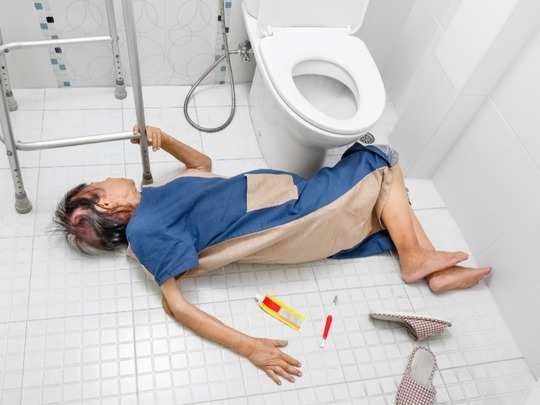Inside a white-tiled bedroom with small square patterns, an elderly woman with black and brown hair is lying on her left side in front of a white toilet bowl. Her left arm, which rests on the floor, clutches a silver walker placed against the back wall. She wears a blue and peach-colored nightgown with a large brown pocket on the front and a blue skirt, while her feet are next to a pair of white and brown checkered slippers. Close to her bottom, there is a yellow tube of toothpaste featuring a red rectangle and a red and white toothbrush. The room is stark with simplicity, accentuated by the white walls, floor, and the visible gray tube from the back of the commode. The woman's posture and vacant gaze towards the wall suggest a state of distress or unconsciousness.